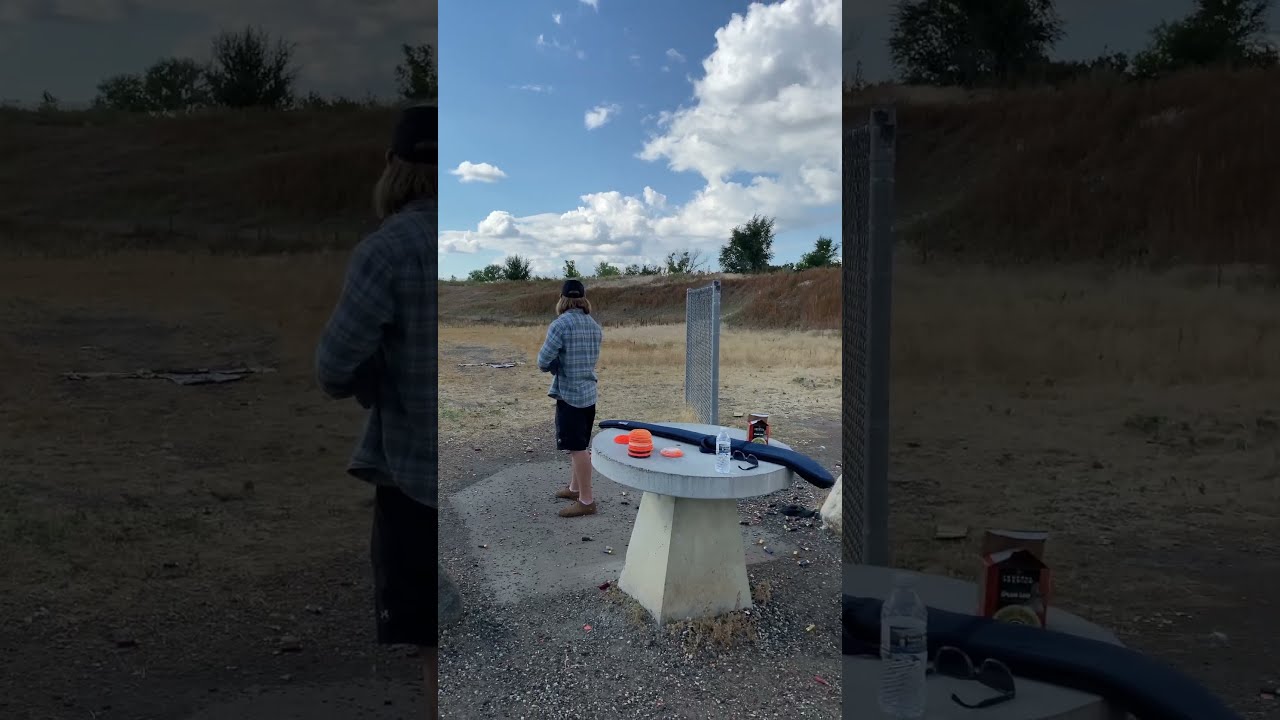In this image, we see a serene outdoor setting under a light blue sky dotted with fluffy white clouds. A man stands on a concrete platform, dressed in a long-sleeve blue plaid shirt, black shorts, brown shoes, and a black baseball cap over his long brown hair. He is positioned near a round, gray stone table with a triangular concrete base, adorned with several orange discs, reminiscent of clay pigeons used in target practice, a plastic water bottle, and a black rifle in a sleeve. The table and man seem to be part of a sparse, open area, hinted at by a single section of chain link fence. The ground around them is patchy with dirt and gravel, and in the distance, green trees frame the horizon. The overall ambiance suggests a calm, sunny day in a somewhat remote spot.